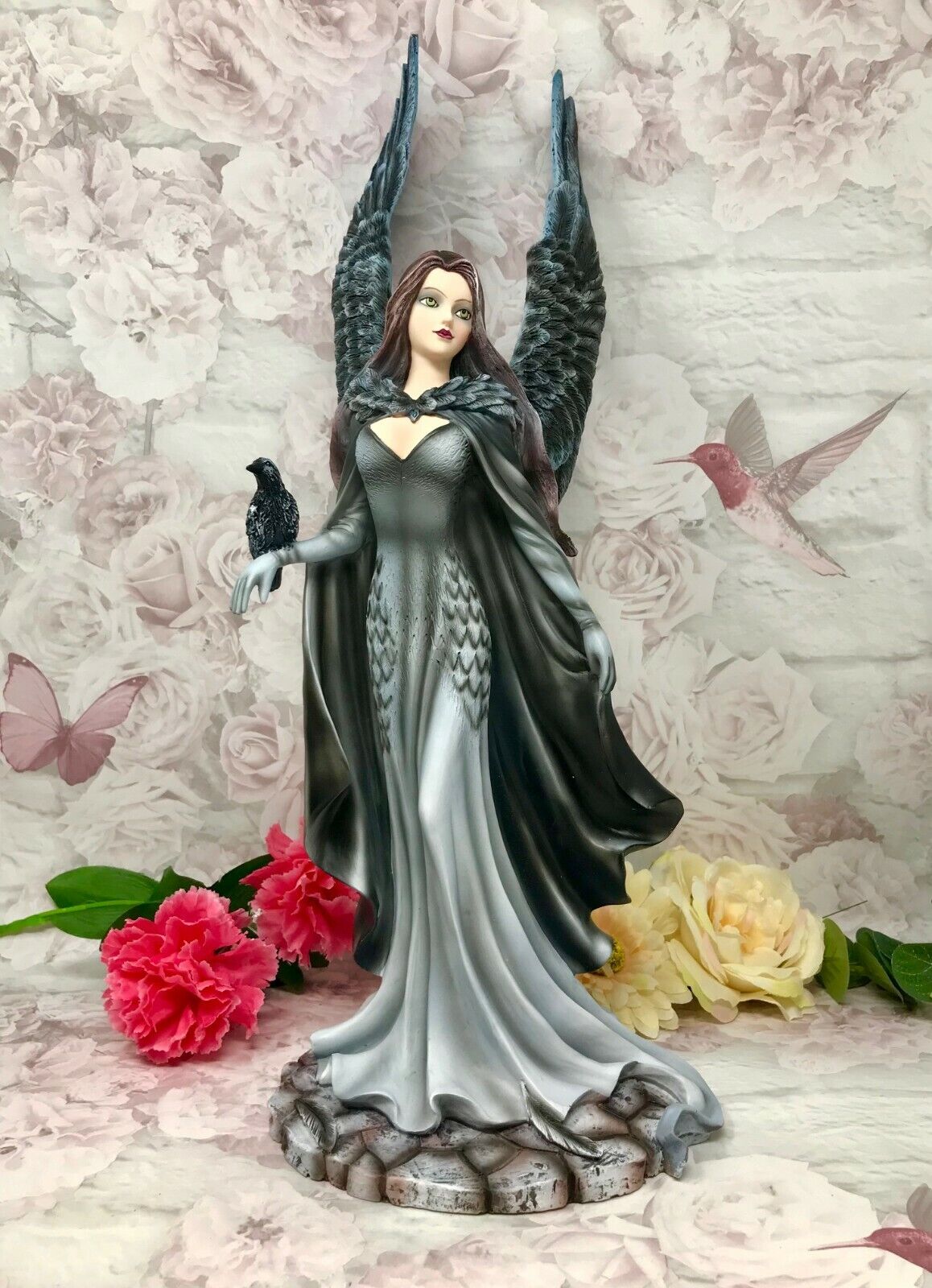The image depicts a highly detailed ceramic sculpture of a young woman with dark, brown hair and black wings, resembling a dark angel. She is dressed in a long, flowing, black and gray dress that extends below her feet and is slightly low-cut, revealing some cleavage. The woman has her right arm outstretched, on which rests a black bird, likely a raven or crow. Her gaze is directed slightly upward and to the right. She stands on a circular stone base, flanked by two red carnations to her left and two yellow roses to her right. The background features a white brick wall adorned with painted hummingbirds, roses, and a butterfly. The combination of the sculpture and the vivid background creates a striking and detailed scene.